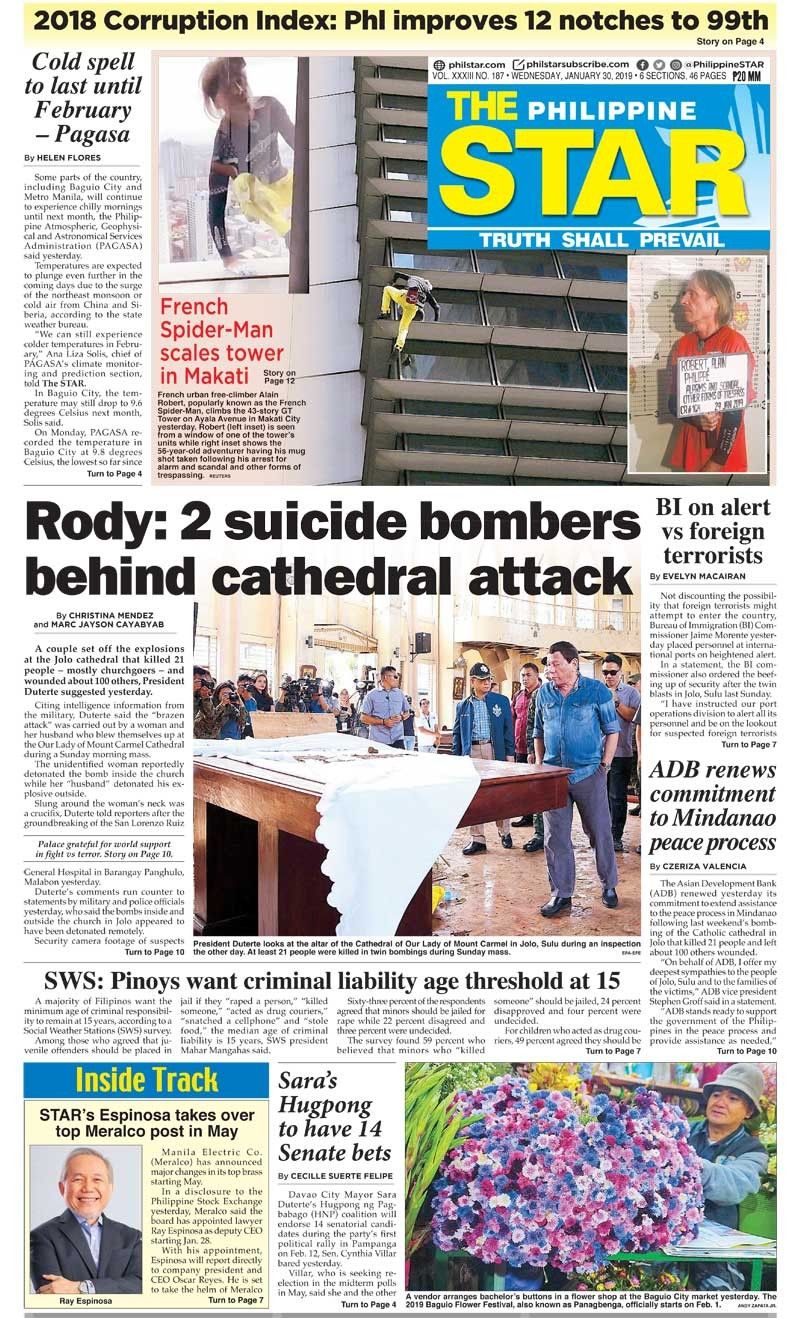The newspaper front page features a prominent headline at the top in black writing that reads, "2018 Corruption Index." Below this, there is an image of a skyscraper with a man in yellow pants scaling the building. A caption in bold red text states, "French Spider-Man Scales Tower in Makati." Further down, there is a mugshot of the same man in an orange jumpsuit, indicating his subsequent arrest.

The next headline, also in black text, reads, "Roddy: Two Suicide Bombers Behind Cathedral Attack." Adjacent to this, there is a photo depicting a group of people standing around a large table, most of whom are men. One man, wearing a blue shirt and gray pants, stands with his hands in his pockets. Another man, positioned behind him, is dressed in a blue shirt, blue jacket, and blue hat.

Towards the bottom, there is a blue rectangle with yellow text that says "Inside Track." Next to this section, there is a picture of a man smiling at the camera, dressed in a gray suit with a blue shirt underneath, crossing his arms.